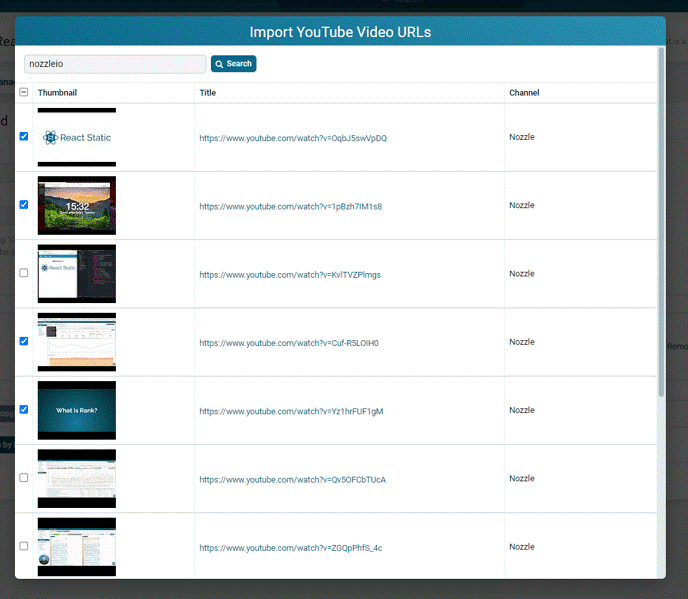The image displays a webpage interface featuring a central square box overlay on a larger, partially visible background website. The central box is distinctive, with a white background and a medium blue ribbon running horizontally across the top. On the blue ribbon, in the upper left corner, the caption "Import YouTube video URLs" is inscribed in white text.

Directly beneath the ribbon, aligned to the left, there is a search bar labeled "Nozzleio" (spelled N-O-Z-Z-L-E-I-O), accompanied by a blue search button. The main content of the box comprises a vertical list categorized into three sections: Thumbnail, Title, and Channel.

The first entry in the list features a thumbnail with the word "React Static" in medium blue text and an accompanying star icon. To the right of this, a snippet of a YouTube webpage is visible, with the associated channel named "Nozzle." This pattern is repeated down the list, and some entries have channels marked with a check mark to their left, indicating they are selected for a specific purpose. The interface combines visual elements of text, icons, and navigation tools to facilitate the import and organization of YouTube video URLs.